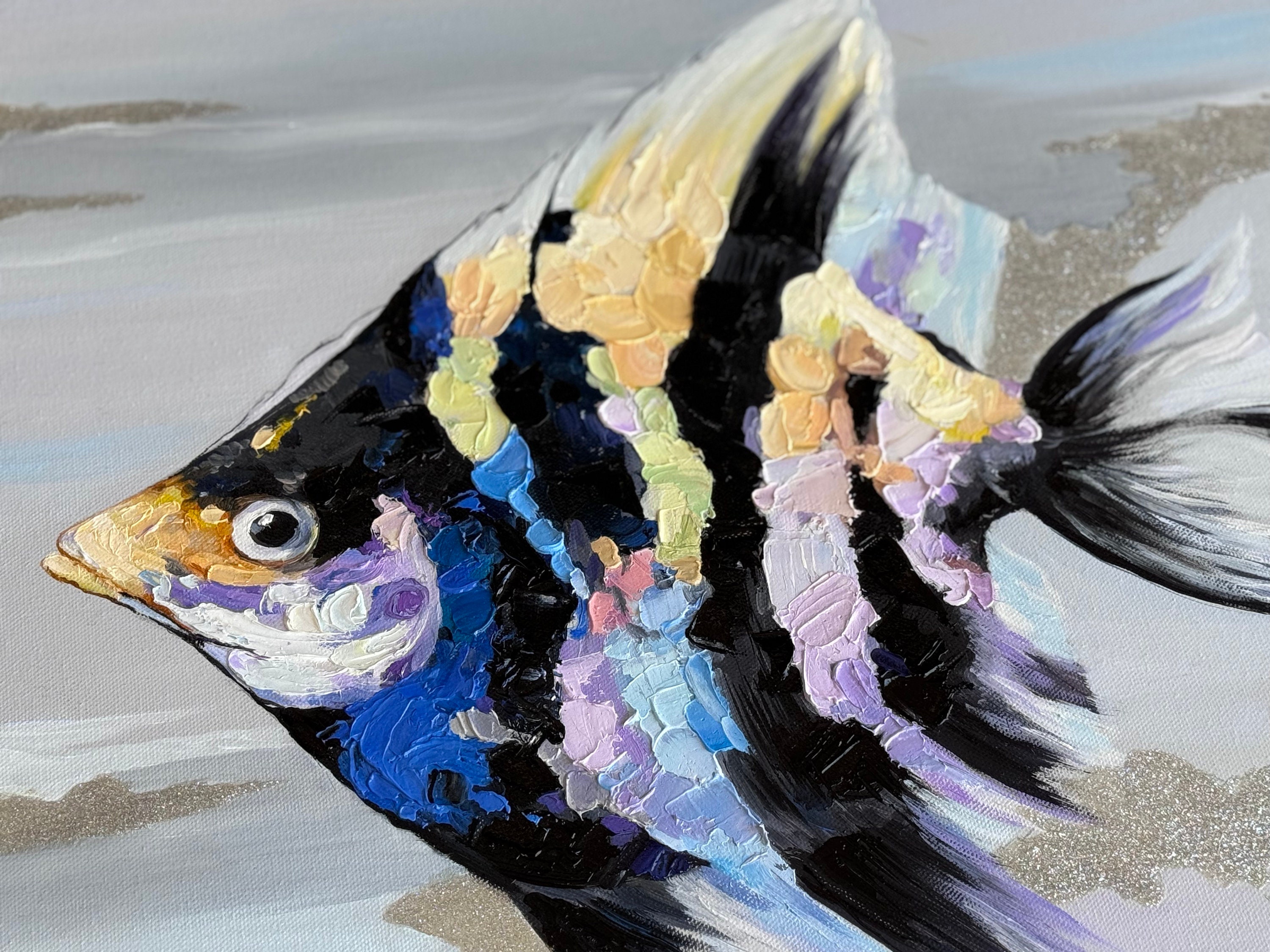The artwork is a detailed painting of a fish displayed on a large square canvas. The fish, which is somewhat triangular or V-shaped, features a head facing to the left and a tail to the right, slightly cropped by the edge of the picture. The fish boasts a color palette of black, blue, purple, white, and gold. Its eye, a realistic depiction, is white with a black center, resembling a wiggly eye with a tiny white dot. The head's top has golden hues, with the mouth appearing golden and the forehead black. At the lower part of the head, white and purple streaks are evident, transitioning into a body decorated in pastel stripes of blue and purple amidst a predominantly black background. The fish's fins extend from top to bottom in an almost triangular shape, with the top fin appearing pointy and golden, while the bottom fin transitions from purple to blue and black. The tail is black, culminating in a white tip. 

The textured background, primarily in shades of white and gray, suggests shallow water, decorated with patches of rocks in the lower right, upper right, lower left, and upper left corners. The area also features white streaks between these rocks, enhancing the aquatic ambiance. Gold accents and glittery touches add depth and a shimmering quality to the composition, suggesting the sunlight reflecting off a watery surface near the shore.